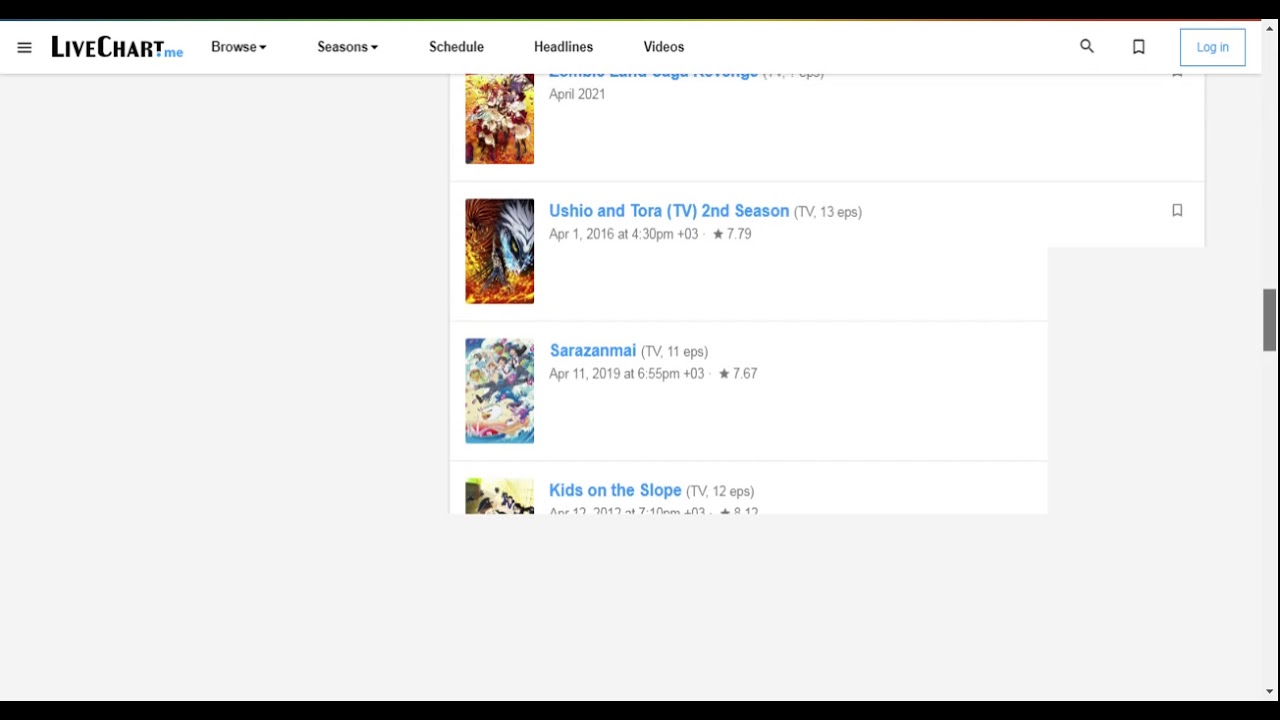The image depicts a web page layout with distinct sections. At the top, there are two black bars—one at the very top and the other at the bottom of the image. Below the top black bar, there is a toolbar that spans across the page. Beginning from the left, the toolbar includes an icon represented by three horizontal lines (typically a menu button), followed by a live chart with "live" displayed in black and ".me" in blue.

Continuing to the right on the toolbar, we see various menu options: "Browse" accompanied by an arrow, "Seasons" with a drop-down arrow, "Schedule," "Headlines," "Videos," a magnifying glass icon indicating a search function, a banner prompting users to save, and a blue square labeled "Login."

Below this toolbar, the main section of the web page is visible, consisting of several segments. The first segment is dominated by three and a half boxes, the first two of which are partially visible. The top half features images with vibrant colors such as red, yellow, purple, and white, though the exact details are indistinguishable. The content is partially obscured, showing only the text "April 2021."

The second segment showcases information about "Ushio and Tora," specifically the TV anime's second season. The details include:
- Title in blue: "Ushio and Tora TV, Second Season"
- Format: TV
- Number of episodes: 13
- Release date: April 1st, 2016 at 4:30 PM (+03:00)
- Rating: 7.79 stars

The next segment features a blue and purple multicolored image with details on "Sarah's Anatomy," including:
- Title in blue: "Sarah's Anatomy"
- Format: TV
- Number of episodes: 11
- Release date: April 11th, 2019 at 6:55 PM (+03:00)
- Rating: 7.67 stars

Following this, there is another segment for "Kids on the Slope," although the bottom line and details are cut off, leaving only:
- Title in blue: "Kids on the Slope"
- Format: TV
- Number of episodes: 12

The detailed captions and descriptions provide a clear view of the web page’s structure and content, albeit with some information partially obscured.